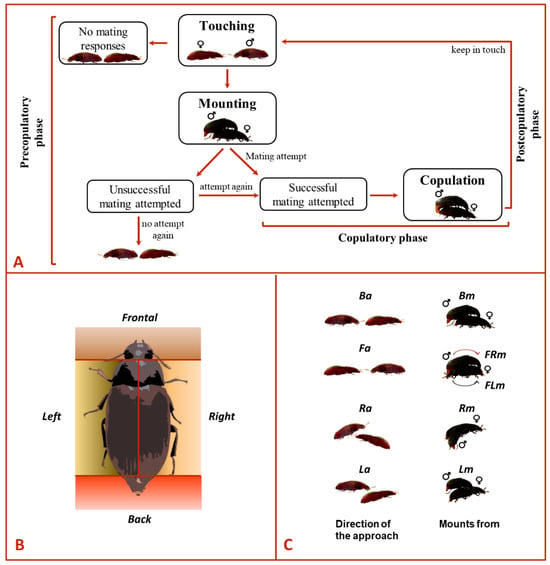This image is an educational chart with a white background and thin red borders dividing it into three distinct sections. The top section, labeled "A" in red text at the bottom left, occupies the upper half of the page, while the bottom half is split vertically into two sections labeled "B" and "C."

The top section, "A," details the pre-copulatory and copulatory phases of some beetle-like insects, possibly roaches. The text "pre-copulatory phase" is rotated counterclockwise on the left side with a red line below it. It illustrates a flowchart starting with a white box with a black-lined border stating "no mating responses," followed by boxes showing subsequent behaviors such as touching, mounting, and mating attempts. If the mating attempt is unsuccessful, the chart indicates an option to attempt again or to document "no attempt again." Successful mating leads to a box labeled "copulation," marking the copulatory phase.

In the bottom left section, "B," there is a detailed depiction of the insect, showing views from multiple angles: frontal (head), left and right (body and legs), and back (tail). This section appears to focus on the insect's anatomy.

The bottom right section, "C," provides images of the insects in different mating positions. It includes labels indicating the directions of approach (Pa, Ra, La) and various mounting forms (BM, FRM, FLM, RM, LM), illustrating how the male positions itself on the female during the copulatory phase.

Overall, this chart provides a comprehensive visual and textual guide to the mating behaviors and anatomical details of the insects in question.